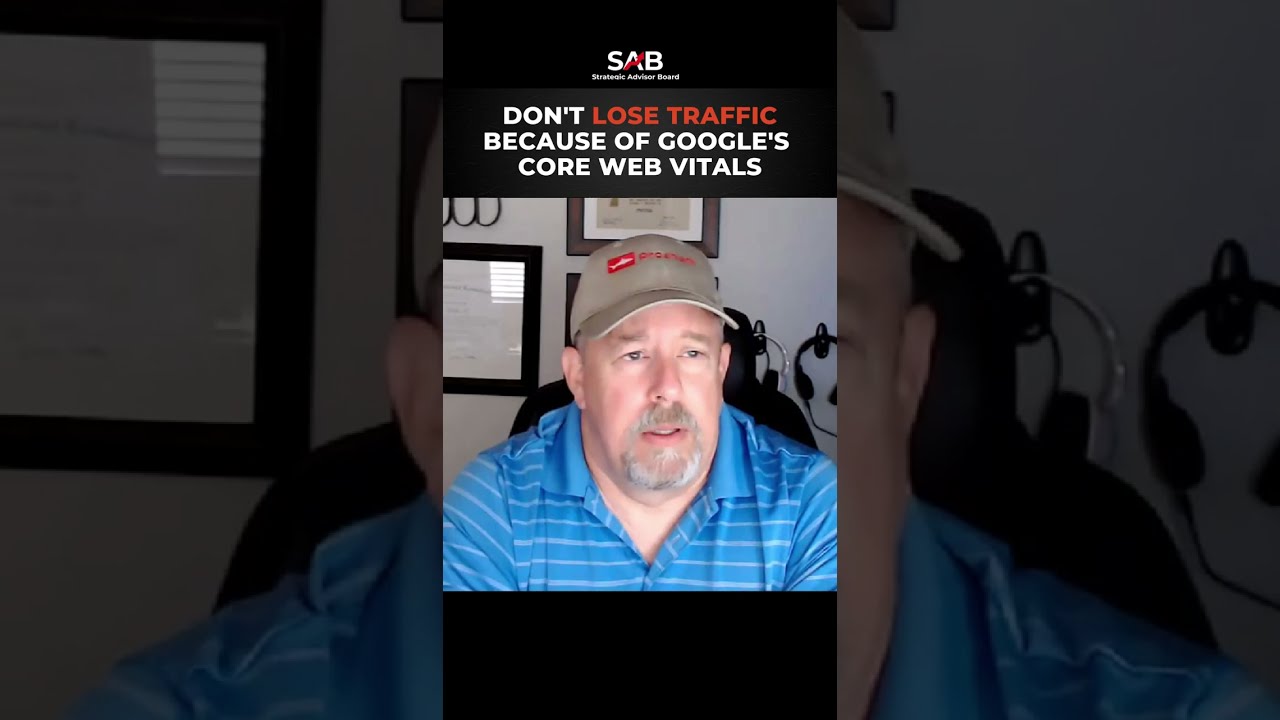In this detailed image, we see a man sitting at a desk in a black chair, wearing a light brown baseball cap with red lettering and a blue short-sleeve polo shirt that features white collars and blue with white stripes. He has a goatee with hints of white and appears to be looking into a screen. Behind him, there are framed credential certificates on a white wall and a pair of headphones. The central photograph, shaped vertically like a smartphone, is prominently placed in the middle of the image and contains a header that reads "SAB." Below it, a text in white states, "Don't lose traffic because of Google's core web vitals," with "lose traffic" highlighted in red.

Flanking the central photo, the background portrays an enlarged, darkened, and slightly transparent version of the same image. This background extends to the left and right, where you can faintly discern parts of his ear on either side, reinforcing that the blown-up image serves as a backdrop. The entire composition resembles the shape of a high-definition television, being wider than it is tall, with black letterboxing at the top and bottom of the central vertical photograph.